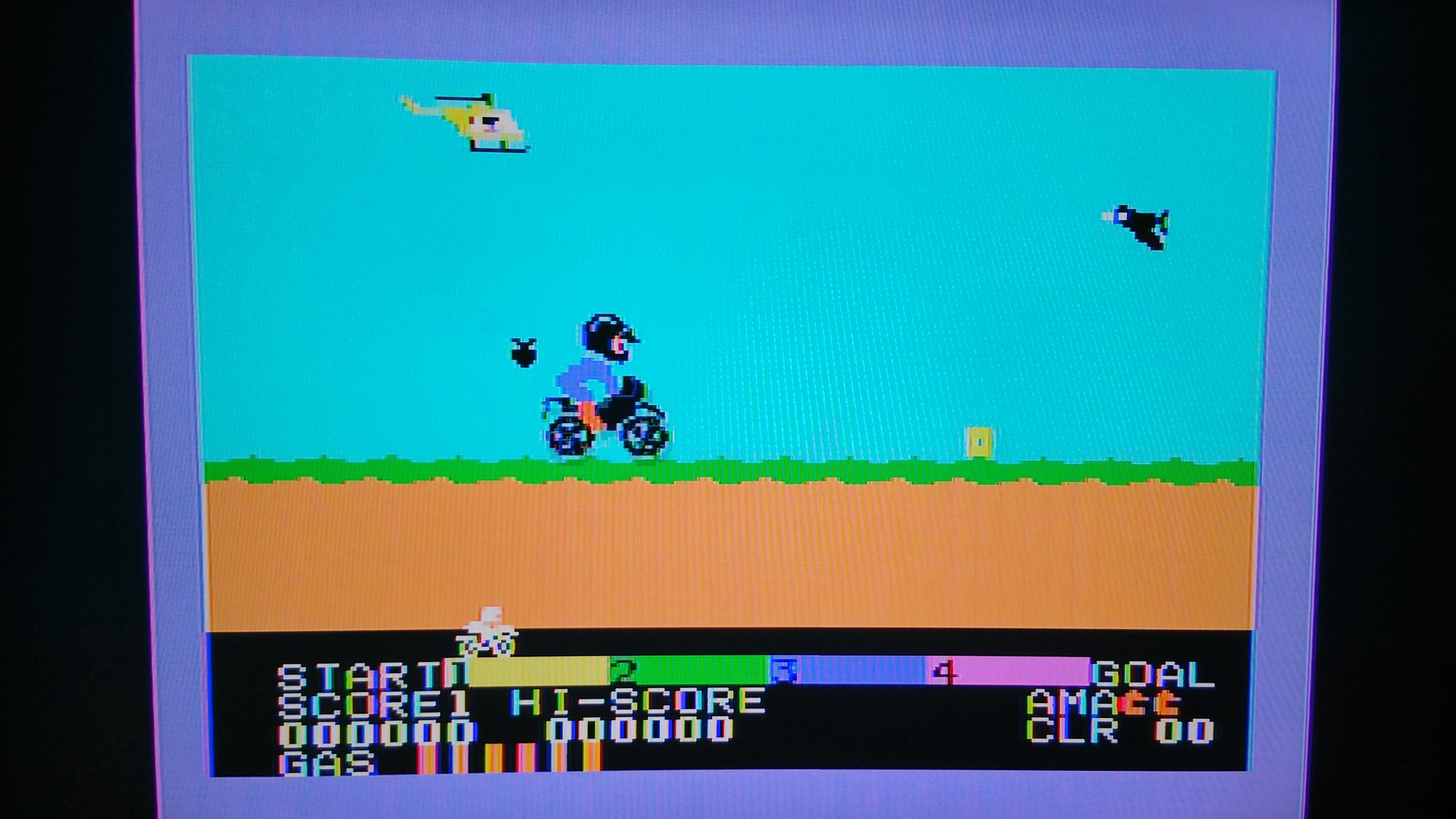The image depicts a scene from an old video game with basic, retro graphics. The central focus is a detailed playable character riding a black motorcycle, donning a black helmet, blue shirt, and orange boots. The motorcycle is positioned on a stretch of green grass, with a thicker brown dirt line beneath it, set against a blue sky. To the left, a yellow helicopter hovers in the air, while a black bird flies to the upper right. The overall scene is framed by a blue border, with black rectangular areas on either side, indicating the picture wasn't large enough to fill the screen. Below, there's a detailed informational display with a "Start" indicator followed by numbered positions in yellow, green, blue, and pink. It also shows a "Goal," "Score," "High Score" with columns of six zeros, two separate times, and a "Gas" meter with six rectangles measuring fuel levels. The display is completed with a "CLR" section and paired zeros.